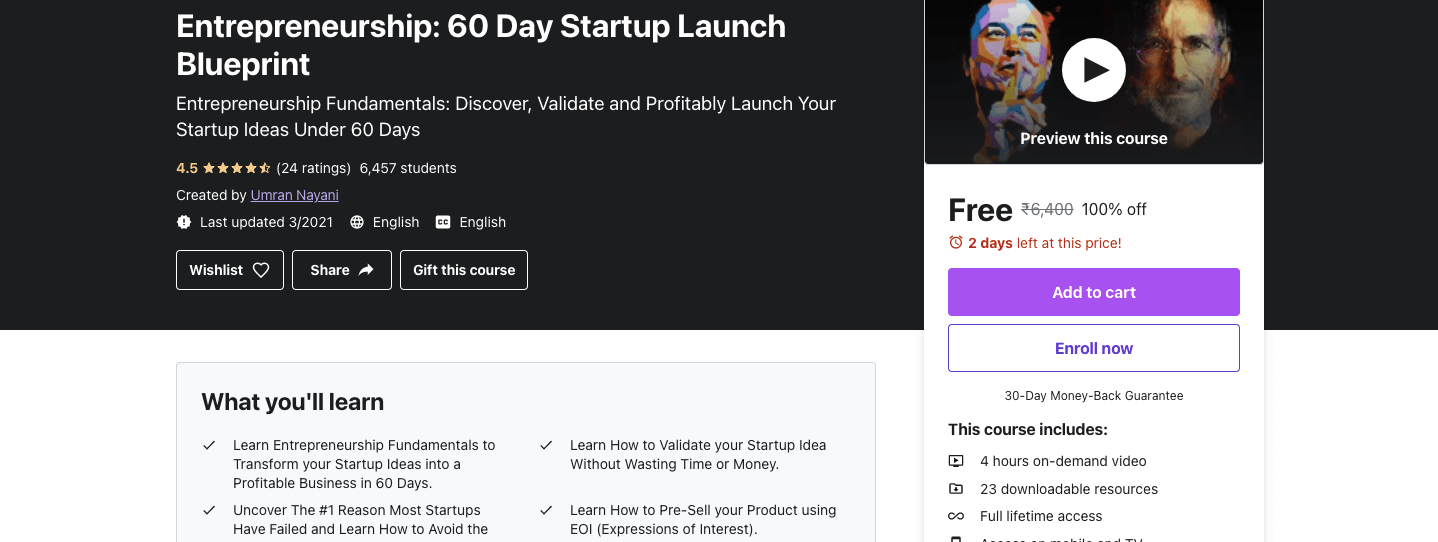**Detailed Descriptive Caption:**

This image is a screenshot of an online course offering page. The layout is divided into two primary sections: the top section features a very dark gray, almost black, background, while the bottom section is white. 

At the top left corner, in large white font, is the title "Entrepreneurship: 60-Day Startup Launch Blueprint." Below this, in smaller white font, it says "Entrepreneurship Fundamentals: Discover, Validate, and Profitability Launcher. Startup Ideas under 60 Days."

Directly beneath this, there is a rating of 4.5 stars based on 24 ratings, presented in white text. It also mentions that the course has been taken by 6,457 students. The creator's name, "Umain Nayani," is listed below, along with the last update date as "3-2021." An icon of a globe indicates the course is available in English, and the "CC" symbol denotes the presence of subtitles.

On the left, there are three interactive options: "Wish List" (with a heart icon), "Share" (with an arrow icon), and "Gift this Course."

To the right, there are images of Elon Musk and Steve Jobs. A play button is placed alongside the text "Preview this course," inviting users to watch a preview. 

Highlighted in large text is "FREE: 100% off," with a note in red, "Two days left at this price." Below, there are two buttons: a purple "Add to Cart" button and a white "Enroll Now" button. At the bottom is a note in small gray font stating a "30-day money-back guarantee." 

In black text, a section titled "This course includes" details the course contents, such as "four hours of on-demand video, 223 downloadable resources," and more. To the left, with a thin blue border, a section titled "What you'll learn" lists key learning objectives related to entrepreneurship.